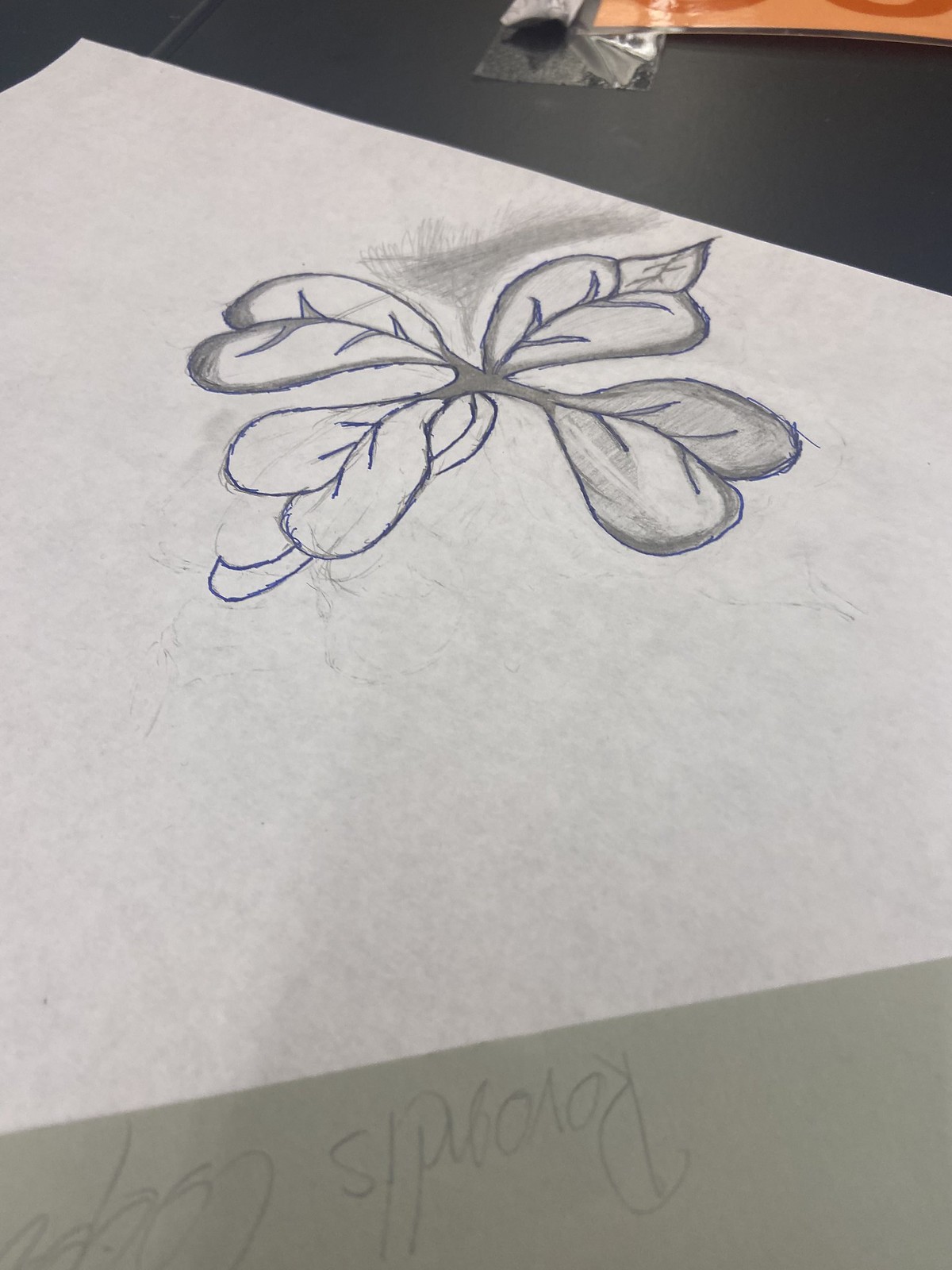A detailed caption for the image could be:

"A detailed drawing of a flower with four petals sits prominently on top of a black desk, which occupies the upper portion of the image. The corner of a piece of saran wrap can be seen intruding from the left, positioned on an orange-hued plastic surface that only partially enters the frame. The flower, the focal point of the composition, is rendered with precision, and an artist's signature is located at the bottom left, extending towards the center. The signature appears upside down. There is also a Byzantium pencil visible in the image, hinting at the medium used for the drawing."